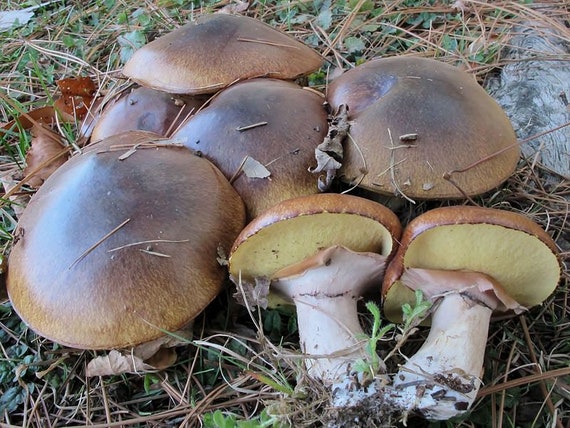In this outdoor, color photograph, a cluster of seven toadstools or mushrooms are nestled in a mixed terrain of dried grass, brown pine needles, and dead leaves, with a flat gray stone visible in the upper right corner. The mushrooms have thick white stems and light brown caps with yellowish rims. Two mushrooms in the bottom right corner lie on their sides, showcasing their pale yellow undersides and creamy edges. These two foreground mushrooms are slightly smaller than the five upright ones still rooted in the ground. The environment appears somewhat dry, with a mix of green and straw-like grass indicating less-than-optimal growing conditions. The mushrooms are all bunched closely together, and some exhibit slight deformations due to their crowded growth.